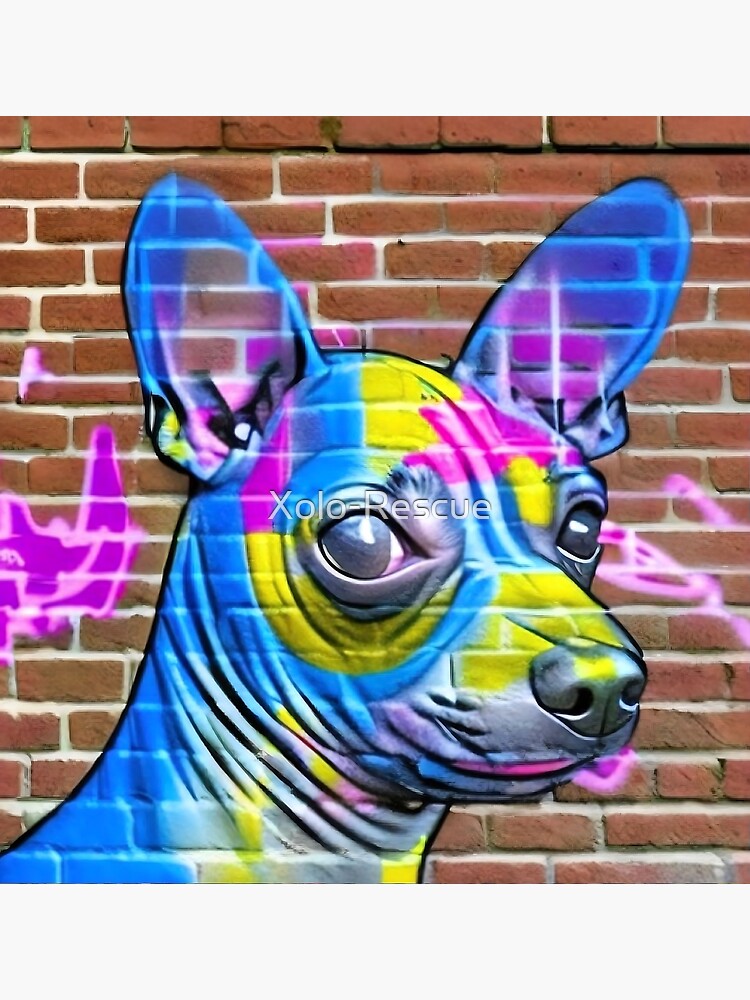The image depicts a digitally constructed, square illustration of a red-brick wall with white mortar lines. Adorning the wall is vibrant graffiti art of a Chihuahua’s head and neck. The Chihuahua's predominantly blue head features intricate color details: yellow splotches below the eyes and on the forehead, pink around the eyes, and a black nose with a gray under-nose area. There are yellow highlights on the lower part of its mouth and neck, which is mostly white with additional yellow streaks. The ears are upright and vividly blue with purple and pink accents. Flanking the dog’s image are pink graffiti tags, and the dog’s design allows the red bricks from the background to show through. The artwork also includes white text in front of the dog that reads “Zolo rescue.”